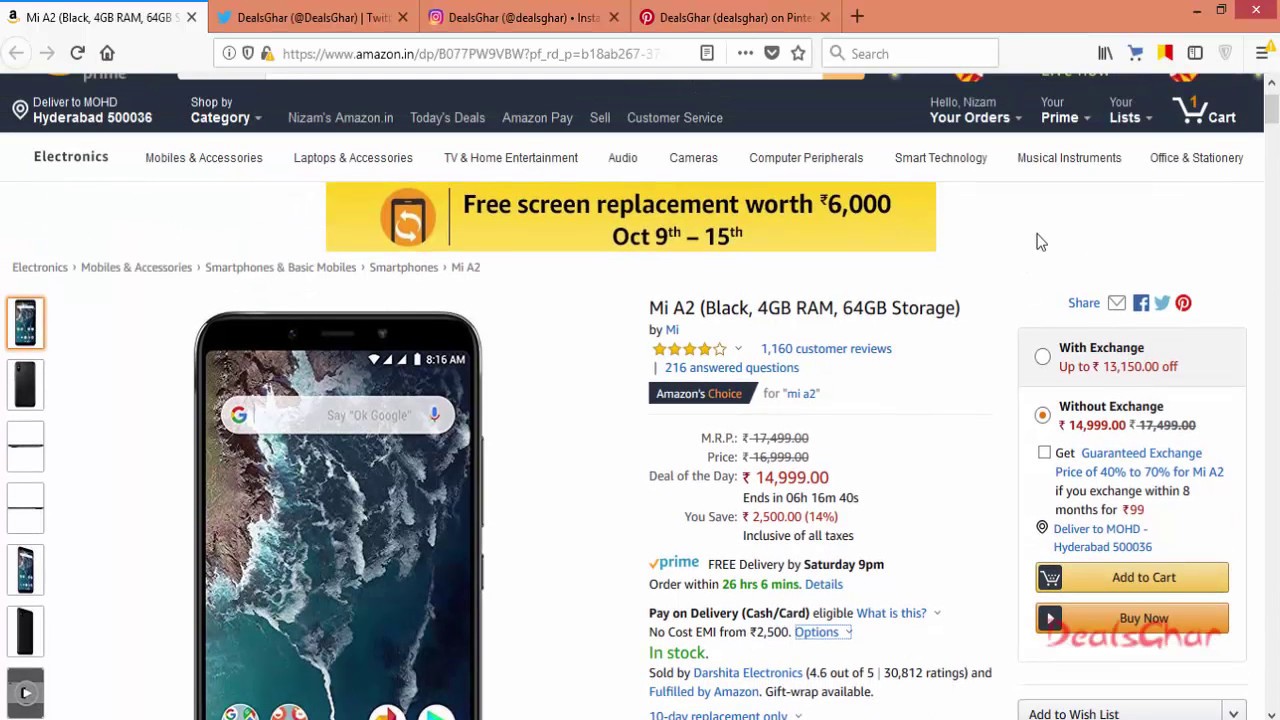This image depicts an Amazon website page viewed through multiple browser tabs. The first tab is white, while the other three are orange. The search bar displays the term "free screen replacement," and an advertisement is prominently featured, marked at $6,000, though the currency unit is unclear, and is valid from October 9th to 15th.

Within the "Electronics" section of the page, a featured item is highlighted: an MI82 black smartphone equipped with 4GB of RAM and 64GB of storage. The phone displays an aerial ocean scene with visible rocks and land. On the left side of the page, there are individual images of the phone, while the right side showcases the Amazon listing details.

The listing, marked as "Amazon's Choice," boasts a rating of four stars based on 1,160 customer reviews. It is advertised as a "Deal of the Day" for $14,999, offering a savings of $2,500, although the currency is not specified. The price is displayed in red text. Free delivery is available by Saturday at 9 PM if the order is placed within the next 26 hours and 6 minutes.

Additional information includes payment options, which accept both cash and credit cards. The listing specifies the seller and mentions options for purchase with or without an exchange. There is a guaranteed discount of 47%, and buttons to "Add to Cart" or "Buy Now" are provided. Handwritten on the page, perhaps digitally, are the words "deals char, C-H-A-R."